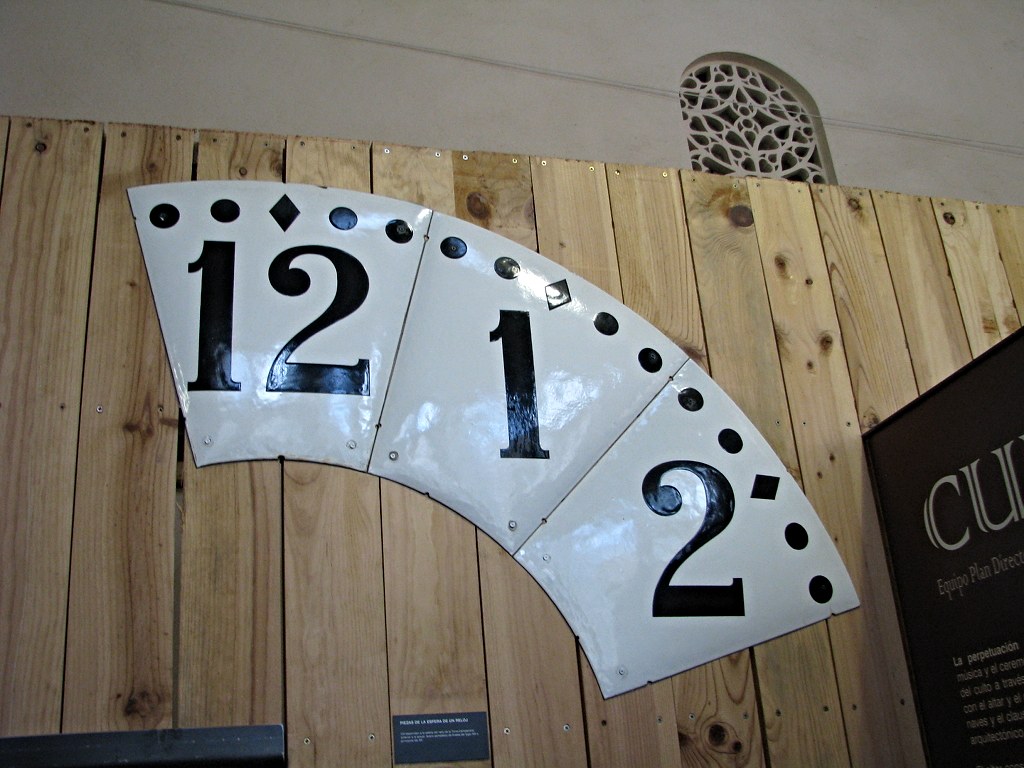The image captures a freestanding wooden wall structure, composed of long, unfinished natural wood boards aligned side by side. Affixed to this structure is a distinctive metal element, shaped somewhat like a quarter-circle or a quarter rectangle. This metal piece is divided into three sections, each featuring a large number and geometric designs against a shiny white background.

The leftmost section prominently displays a large black number '12' on a white square. Above this number, there are four circles, with a diamond shape positioned in the middle, flanked by two circles on either side. The middle section mirrors this geometric arrangement, with a number '1' below the pattern of circles and the diamond. The rightmost section also features the four circles and diamond design, with the number '2' beneath them.

In the background, at the top-right corner of the image, an ornate, small window suggests that the setting could be part of the exterior wall of a building, possibly a church. Below the metal element, there is a small label attached to the wooden wall. Visible screws secure the wooden slats in place, adding to the rustic, unfinished appearance of the structure.